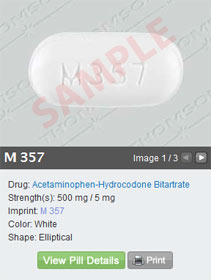This detailed screenshot captured from a medical or pharmacy-related website provides a comprehensive overview of the drug M357, also known as acetaminophen and hydrocodone. The listing includes two strength options for the medication: 500 mg of acetaminophen and 5 mg of hydrocodone. The pill, identifiable by its M357 imprint, is white and elliptical in shape. The interface prominently features a green button for accessing more detailed information about the pill, alongside a print button and options for viewing three different images of the medication. Acetaminophen is categorized as a pain reliever, while hydrocodone is recognized for its potent analgesic effects. This page appears to be designed for use by pharmacies or medical professionals, providing essential physical and pharmaceutical details about the pill to ensure proper identification and understanding of its uses and manufacturing variations.